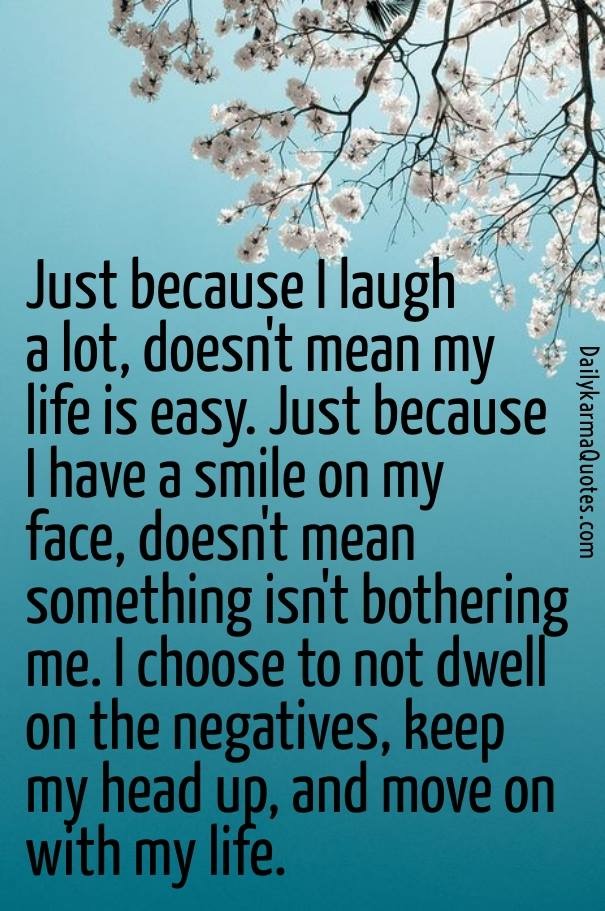The image features an inspirational poster with a gradient blue background, transitioning from a dark blue at the bottom to a lighter blue at the top, resembling a sky. In the upper right corner, delicate tree branches adorned with white cherry blossoms, some with pink centers, add a touch of natural beauty. Below the floral imagery, a powerful quote is displayed in large, bold black lettering: "Just because I laugh a lot doesn't mean my life is easy. Just because I have a smile on my face doesn't mean something isn't bothering me. I choose to not dwell on the negatives, keep my head up, and move on with my life." Additionally, the poster includes the text "dailykarmaquotes.com" written in black, oriented vertically along the side from top to bottom.